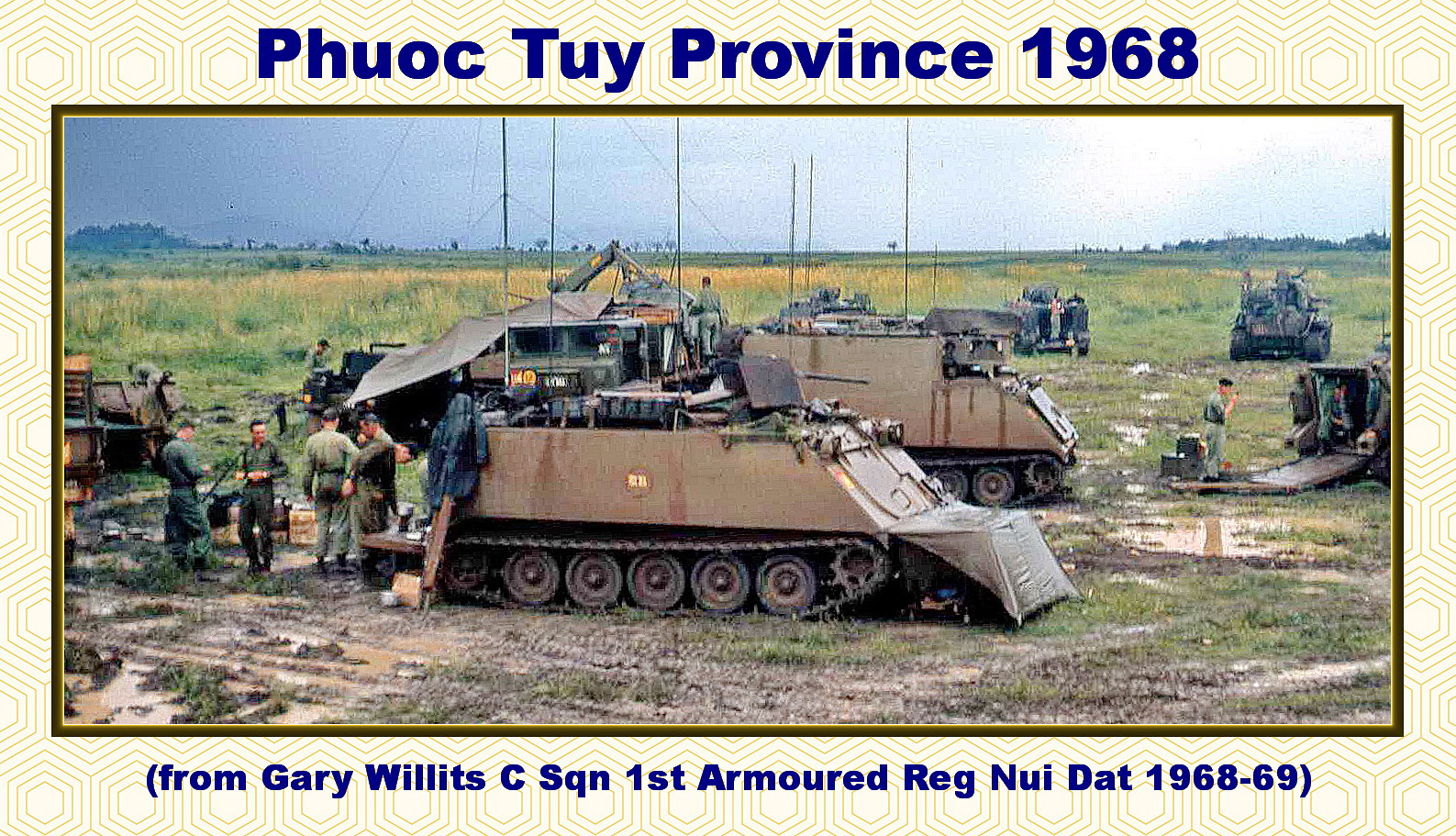The photograph, rectangular and wider than it is tall, depicts a scene from the Vietnam War, specifically Phuoc Tuy Province in 1968, as indicated by blue text at the top. The image is framed by a border with hexagonal patterns and a faint white or greenish hue. At the bottom, it notes, "From Gary Willits, C-Squadron, 1st Armored Regiment, Nui Dat, 1968-69."

The central focus shows a military setup in a muddy, brown-watered field. In the foreground on the right, a light brown troop carrier with treads and raised antennas sits near a tent-like structure. Behind it, another troop carrier can be seen with various track vehicles and supporting equipment around it. Further in the distance, additional vehicles include trucks and what appears to be an excavating machine.

Near the front troop carrier, soldiers in light green uniforms go about different activities, with one possibly holding a cup of coffee. There's an awning-like structure at the back of the carrier and a green material visible behind it. On the left, another vehicle, perhaps a Jeep, has a man inspecting its interior.

In the midground, a troop carrier with its rear open reveals a man speaking into a radio, accompanied by transmitting equipment. To the upper right, a tank points its muzzle rightward, topped by a machine gun. The landscape features a mix of dirt and grass, leading up to a horizon line punctuated by trees under a gray, patchy sky.

This scene captures what seems to be a communication center with soldiers and vehicles stationed in a tactical assembly, their antennas raised, poised for further action amidst the conflict of the Vietnam War.